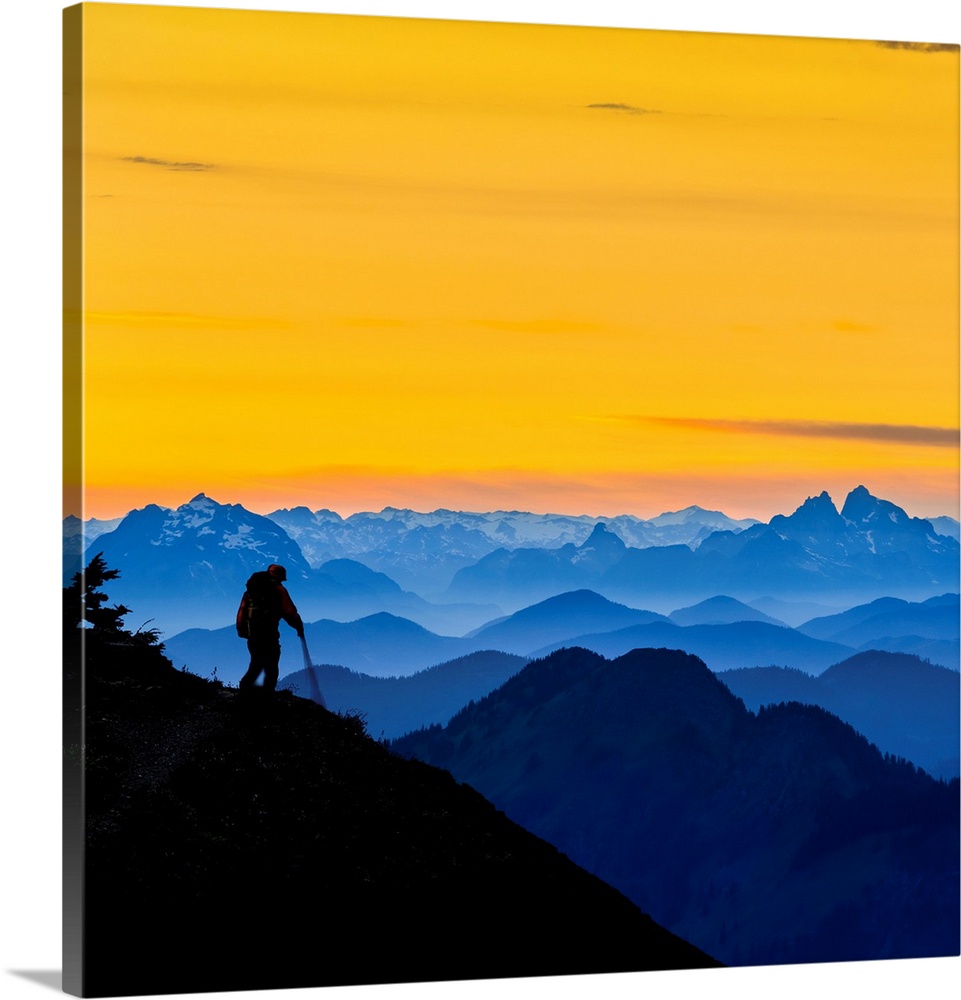This artwork depicts a vivid, painted scene dominated by a golden-yellow sky streaked with dark lines, suggesting either a setting sun or an artistic interpretation of twilight. The foreground features a stark black hill where a lone hiker, silhouetted in black, manages a steady descent while leaning on a hiking stick and carrying a backpack. The midground showcases an indigo mountain, adding depth to the composition, while the background unfolds into a series of blue mountains, some capped with snow or ice, extending into the horizon. The entire scene is set on a platform, resembling a square tablet with noticeable thickness, enhancing the visual impact of this striking, graphic landscape.